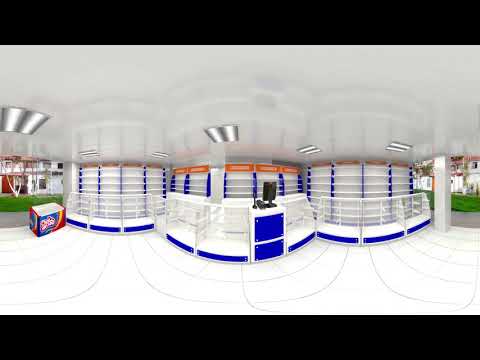The image depicts a panoramic 360-degree view of what appears to be an empty storefront or a movie set designed with a futuristic theme. The store has three prominent circular shelving units, each white with blue trim, giving an impression of doorways or columns but are in fact functional shelves without any items on them. There's a central counter that is also circular, featuring a monitor facing away from the viewer. To the left, there's a colorful box—showing hues of orange, red, and blue—placed near one of the shelving units on the floor, though its contents are indiscernible. The floor is predominantly solid white, accented by silver and blue lines, while the reflective white ceiling is dotted with light fixtures. Outside the open sides of the structure, green hedges, trees, and distant shops can be seen, adding to the enclosed yet open atmosphere of the scene.